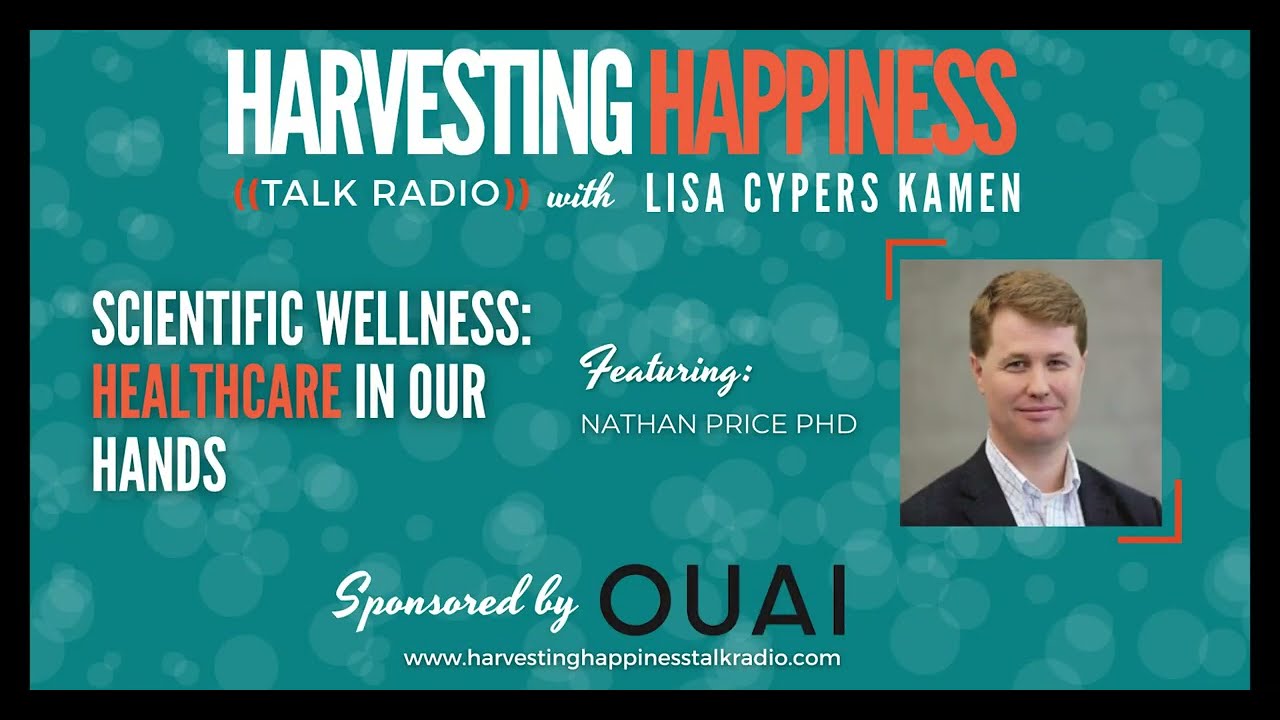This digital business card-style landscape image, potentially an advertisement for a podcast or radio show, features a medium green-blue background adorned with white bubbles or circles. At the top, the title "Harvesting Happiness" stands out with "Harvesting" in white text and "Happiness" in orange text, followed by "Talk Radio" in white text enclosed by orange parentheses, all together with "with Lisa Cypress Kamen" in cursive. The central portion of the image highlights "Scientific Wellness Healthcare in our Hands," with "Healthcare" in orange text. To the right, it features "Nathan Price, Ph.D.," accompanied by a portrait of a smiling gentleman in a black suit and white shirt, set against a tan background. At the bottom, the image indicates that it is "Sponsored By" OUAI in large block letters, followed by the website "www.harvestinghappinesstalkradio.com" in white text.